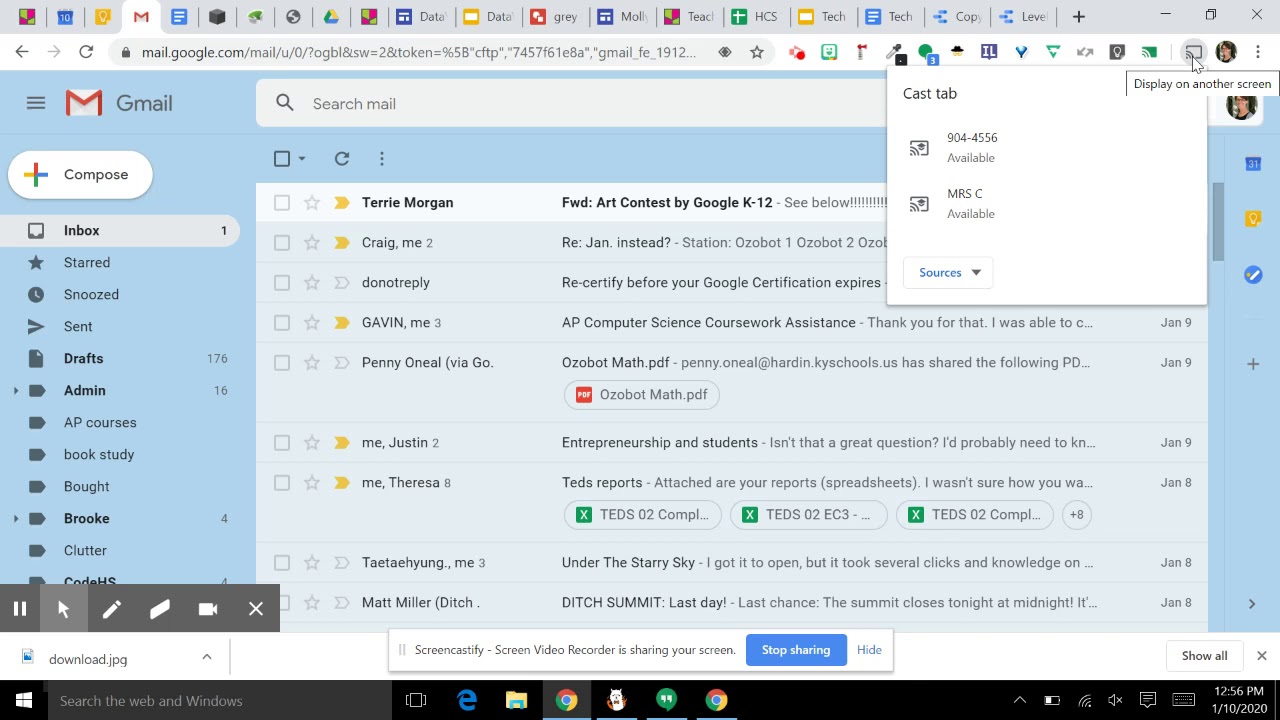The image shows a computer screen with multiple browser tabs open at the top, focusing on one particular tab displaying Google Mail. There's a blue background with a gray inbox area in the center, indicating the selected "Inbox" section on the left-hand options panel. The user has one new message, which is from Terry Morgan with the subject "Forward: Art Contest by Google K-12, see below."

At the top of the inbox, there's a mail search bar. In the upper-right corner of the screen, there is a white pop-up window labeled "Cast Tab," which contains two options: "904-4556 available" and "Mrs. C available." There's also a drop-down menu labeled "Sources."

At the bottom of the screen, a white notification bar indicates that "Screencastify - Screen Video Recorder is sharing your screen," accompanied by a blue "Stop sharing" button.